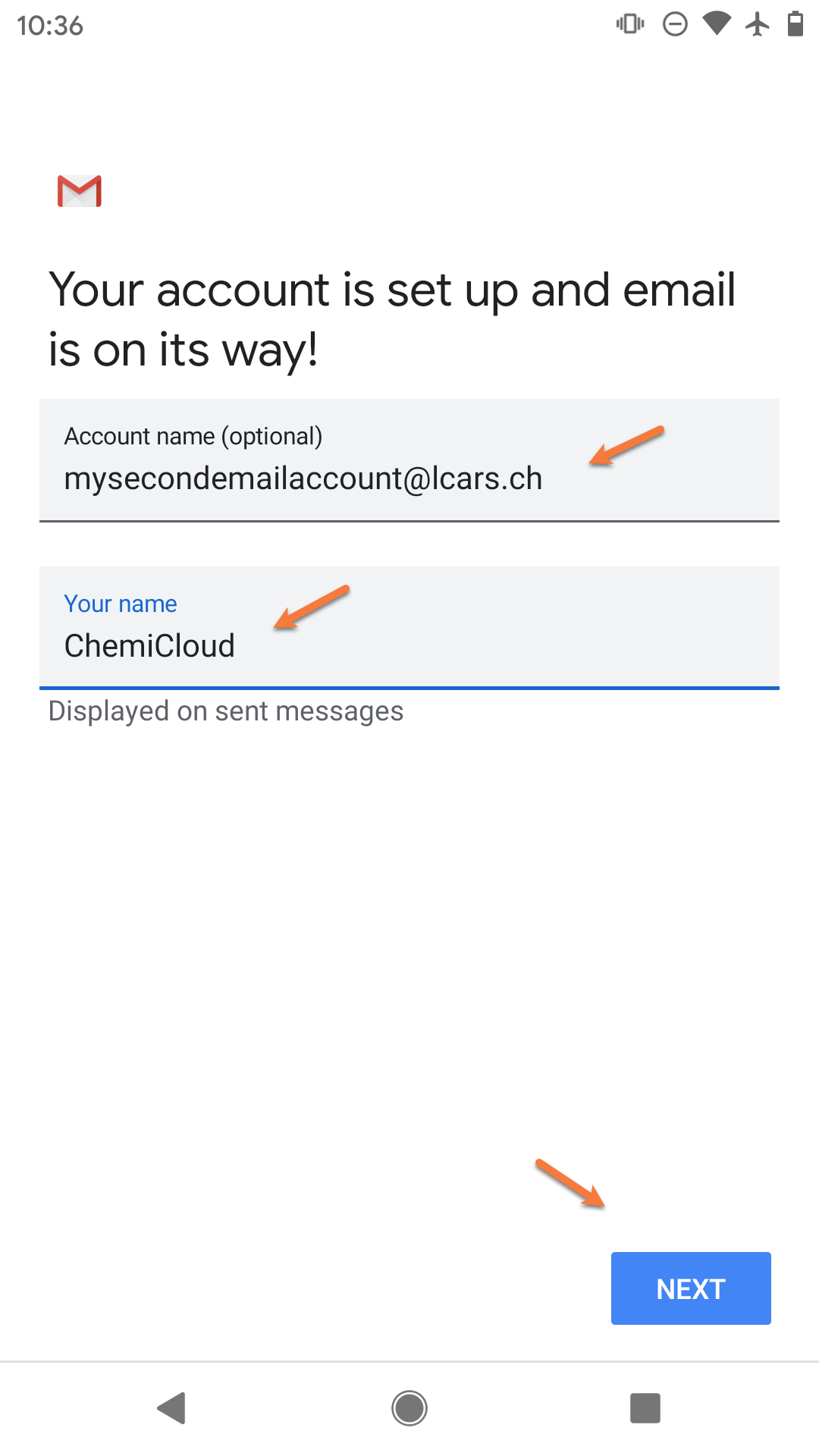This is a detailed screenshot taken from a cell phone, set against a completely white background with dark gray or black text throughout. In the upper left corner of the image, the timestamp reads 10:36. The status icons to the right indicate that the phone is at approximately 50% battery, in airplane mode, with Wi-Fi grayed out, and in 'Do Not Disturb' and vibration modes.

Moving to the top left of the screenshot, the familiar Gmail icon, characterized by a white envelope with red envelope lines, is visible. Underneath, the text reads: "Your account is set up and email is on the way." Below this statement, there is a form field labeled "Account name (optional)," which has been filled in with the email address "mysecondemailaccount@lcars.ch."

A noticeable red arrow points to this email address, emphasizing the "account name" field (albeit filled with an email instead of a name). Another red arrow directs attention to the "Username" field, which reads "KimmyCloud" (stylized as CHEMICLOUD in one word). Toward the bottom of the screenshot, a third red arrow points to a blue "Next" button, indicating the subsequent step in the process.